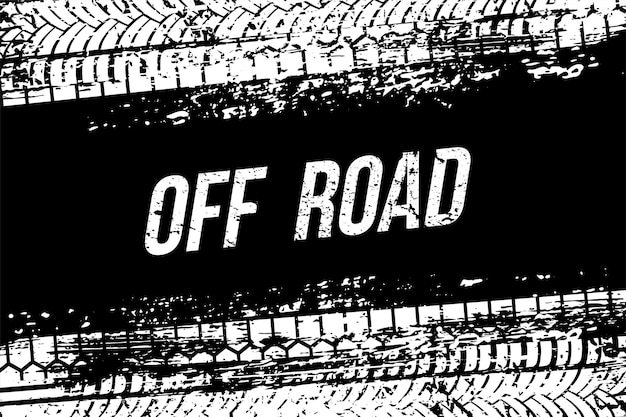The black-and-white illustration prominently features the phrase "OFF ROAD" in bold, italicized, all-capital white letters with a speckled black pattern within the font, situated centrally on a diagonally oriented black strip. Tire tread marks, characterized by their white coloration interspersed with black outlines, traverse both the top and bottom portions of the image, aligning diagonally from the top left towards the top right and vice versa. The overall aesthetic, including the distinctive tire tracks and bold lettering, suggests it is likely an advertisement or signage related to off-road racing.